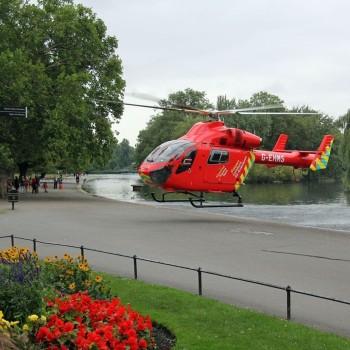The image captures a vibrant outdoor scene centered around a bright red helicopter with yellow and blue accents, marked with the letters G-EMMS on its tail. The helicopter’s spinning blades suggest it is either landing or taking off, hovering just a few feet above a smooth, light gray paved surface, likely a walking path in a park. Surrounding the main scene are well-kept patches of green grass, vibrant flower beds containing a riot of colors including yellow, gold, orange, purple, and bright red flowers, possibly poppies, all enclosed by a low fence. In the backdrop, there is a tranquil body of water, possibly a lake, with trees lining the background. Additionally, some people can be seen walking and gathering near a garbage can under the trees to the left, while a small ripple effect is visible on the lake to the right due to the helicopter's motion. The scene is set under a clear blue sky, enhancing the sense of a bright, sunny day.